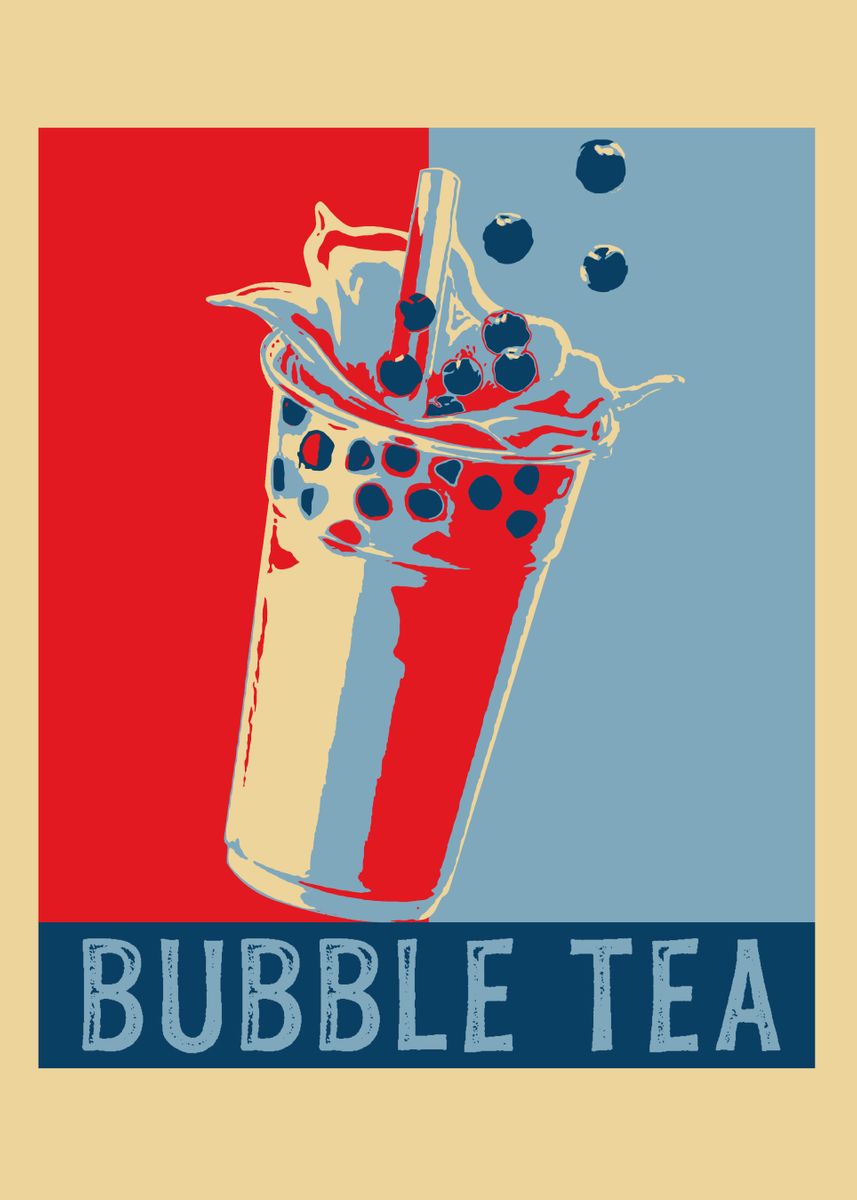An illustration inspired by the iconic "Hope" poster from President Obama's campaign prominently features the familiar split-color scheme of reds and blues. The background has a tan hue with vertical stripes dividing it into two halves: one blue and one red. In the center of the image is a plastic container of bubble tea, complete with a straw and the signature tapioca pearls at the bottom. Beneath the cup, the words "Bubble Tea" are proudly displayed, mimicking the stylistic typography of the original "Hope" artwork. The overall composition creatively blends pop culture with a nod to a memorable piece of political art.